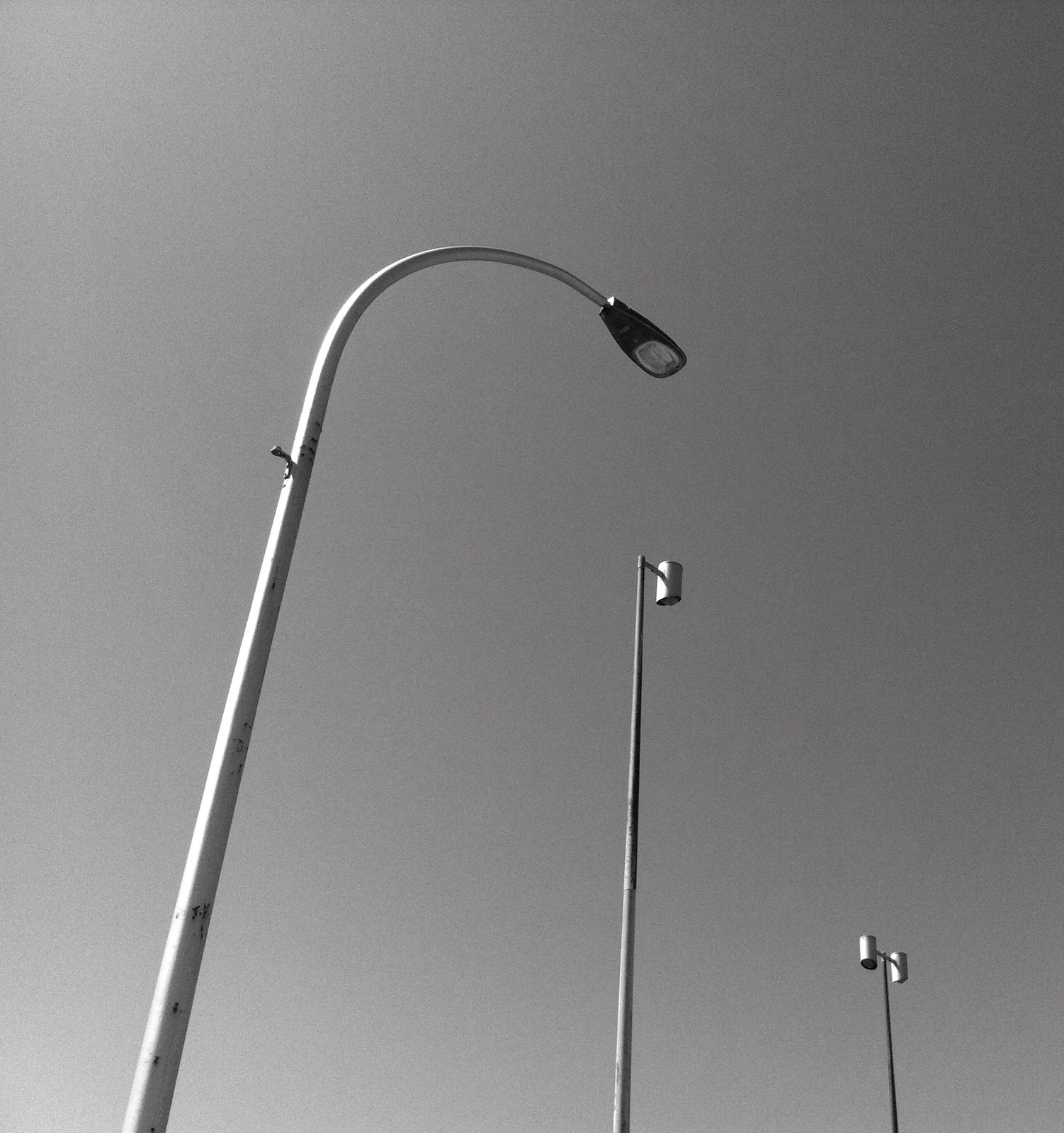This outdoor black and white photo captures the perspective of someone standing on the ground, looking up at three light poles against a contrasting gray sky. The foremost light pole emerges from the lower left-hand corner, characterized by its sleek, silver design that curves at the top. It features a black metal housing for a sizeable spotlight, casting light downward. Positioned centrally, the second light pole stands tall and straight, ending in a single, box-shaped light fixture that also illuminates the ground below. The furthest pole, located in the lower right-hand corner, appears smaller due to distance. It has a straight central shaft supporting two symmetrical, box-like light housings, one on each side. This minimalist composition emphasizes the stark geometric shapes of the poles and light fixtures against the varying shades of the gray sky.